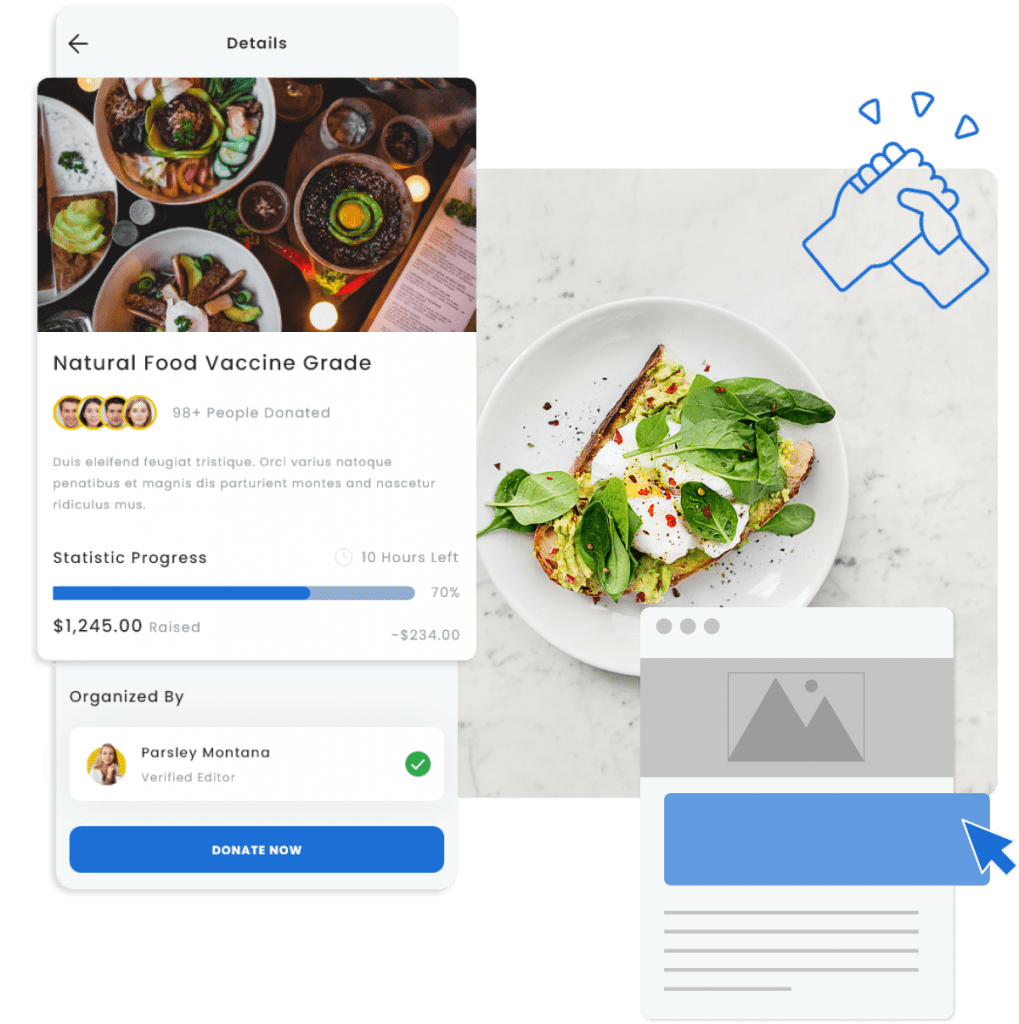The image is divided into four distinct panels. The first panel, situated on the left, features a light gray background with a black arrow pointing left. Centered within the panel is the word "Details" in bold, capitalized letters. Above this is an overlaid section that displays an aerial view of various plates and bowls of food, showcasing a variety of sizes—larger bowls, smaller bowls, and accent pieces containing condiments.

Below this image are the words "Natural Food Vaccine Grade," with each word's initial letter capitalized. Beneath this text, there are small circular images representing different individuals, accompanied by the phrase "98+ people donated." There is additional text in a different language followed by "Statistic Progress" in black print, indicating "10 hours left." A blue progress bar beneath this shows that the donation goal has reached 70% completion, with $1,245 raised out of the total needed, which is $1,479, leaving $234 still required. At the bottom, it is indicated that the initiative is "organized by Parsley Montana, Verified Editor," with a "Donate Now" button prominently displayed.

The right side of the image showcases a delectable plate of avocado toast topped with an egg and greens, with two hands clasped together in a graphic. Above this, there is a floating pop-up with a white border top and graphics resembling mountains with a blue background below them.